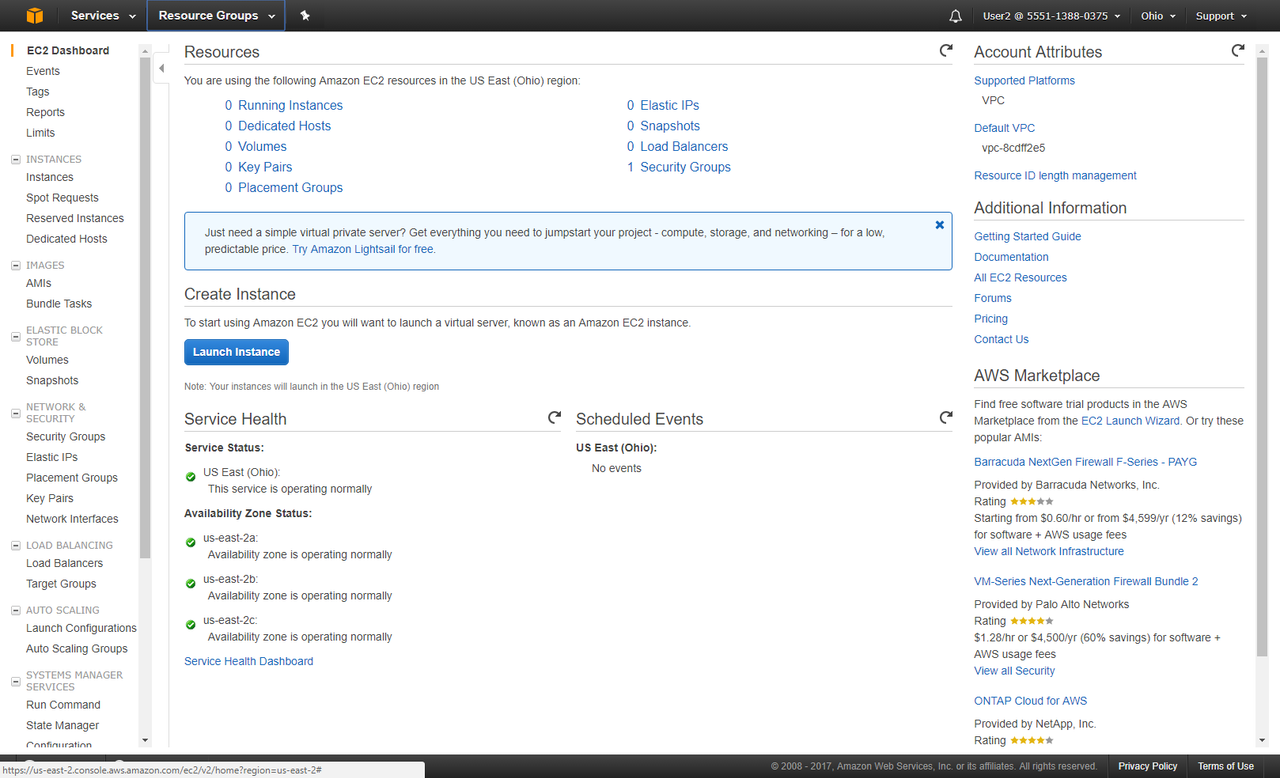The image is a screenshot from a software interface displaying various Amazon EC2 services and resource groups. At the top of the interface, there is a navigation bar with the labels "Services" and "Resource Groups." To the right on this bar, there is a bell icon for notifications, along with an identifier showing "User 2 at 5551-1388-0375 in Ohio," and an option for support.

On the left-hand side, a vertical column lists various sections:
- **EC2 Dashboard**: including options like Events, Tags, Reports, and Limits.
- **Instances**: with sub-options such as Instances, Spot Requests, Reserved Instances, and Dedicated Hosts.
- **Images**: allowing choices between AMIs or Bundle Tasks.
- **Elastic Block Store**: offering options like Volumes and Snapshots.
- **Network & Security**: featuring choices such as Security Groups, Elastic IPs, Placement Groups, Key Pairs, and Network Interfaces.
- **Load Balancing**: with options for Load Balancers and Target Groups.
- **Auto Scaling**: where you can configure Launch Configurations or Auto Scaling Groups.
- **Systems Manager Services**: including options for Run Command, State Manager, and Configuration.

The main part of the screen outlines the resource usage for Amazon EC2 in the US East (Ohio) region. The resources in use include:
- Running Instances
- Dedicated Hosts
- Volumes
- Key Pairs
- Placement Groups
- Elastic IPs
- Snapshots
- Load Balancers
- One Safety Group

Below this section, there are options to create and launch instances. Additionally, the Service Health section indicates the status of various services:
- US East (Ohio) is operating normally.
- Availability Zone Status shows:
  - US East 2a: Operating normally
  - US East 2b: Operating normally
  - US East 2c: Operating normally

Lastly, there are options to access the Service Health Dashboard and view Scheduled Events, with the information that currently, there are no events in the US East (Ohio) region.